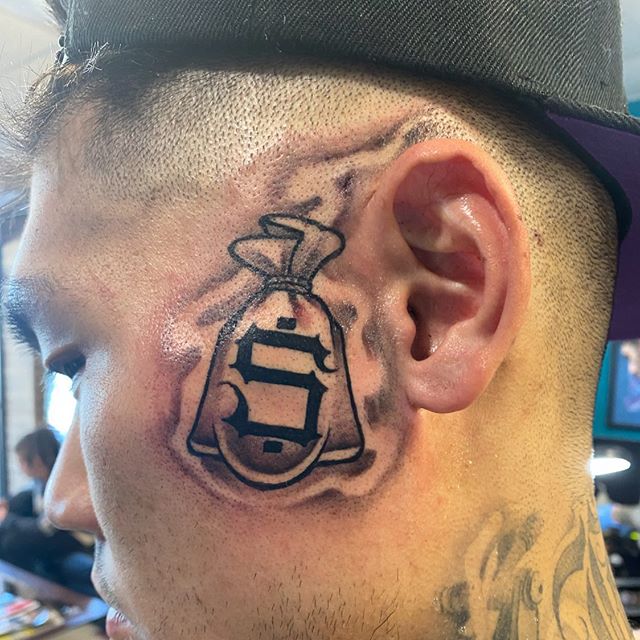This close-up photograph captures an Asian man with a partially shaved head and very short hair above his forehead, wearing a black baseball cap turned backwards. Dominating the image is a conspicuously large and fresh black tattoo near his left ear and down his neck. The tattoo in front of his ear features a detailed bag of money with a prominent dollar sign. The skin around it appears red and swollen, indicating it was recently done. His unshaven face reveals small hair stubble, and another indistinct black tattoo is visible on the back of his neck. The man is looking down, and in the blurry background, there are indistinguishable figures in a room, adding context to the indoor setting. His skin tone is peach-colored, and he appears to have a serious expression.